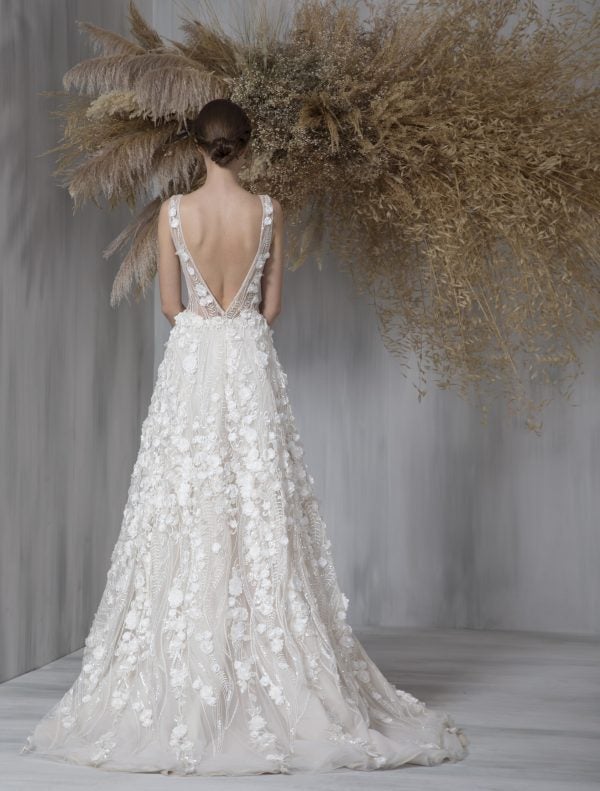The image depicts a woman, likely on her wedding day, standing on the left side of the frame with her back to the viewer. She is dressed in an exquisite, long, white wedding gown that drapes elegantly onto the floor. The backless dress has a deep V-cut down to her waist and is adorned with intricate white floral designs made from ornate material sewn onto a delicate veil-like overlay. Her hair, a rich dark brown, is styled neatly in a bun, exposing her light skin. She stands in a gray-walled room with matching gray flooring, facing a corner. In front of her is a large, dried, puffy plant with reddish-brown tones that adds an additional textural element to the neutral surroundings.